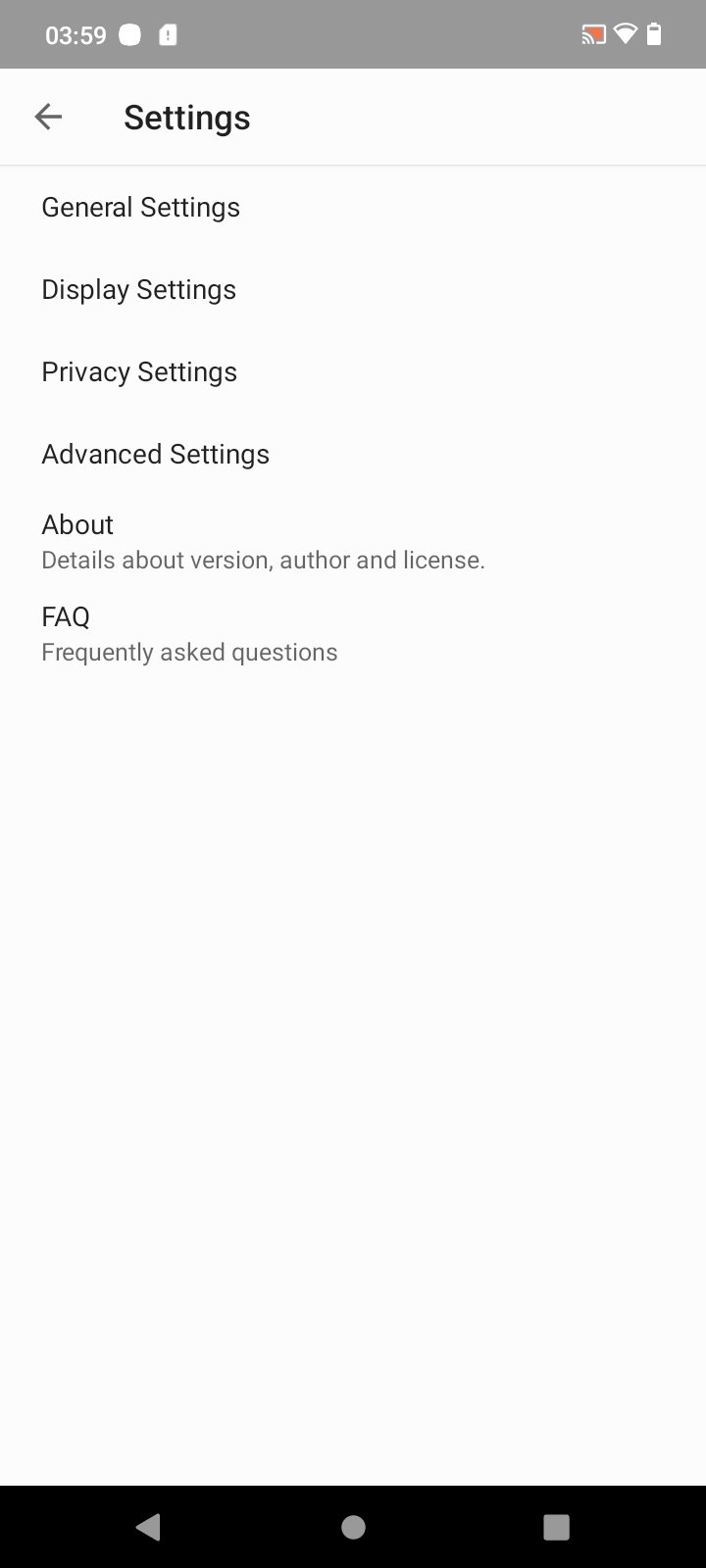The image features a screenshot of a smartphone's settings menu. At the top, a dark gray border contains a smartphone icon, the time displayed as 3:59 on the left, and Wi-Fi and battery icons on the right. Below this border, the background is a very light shade of gray.

Directly beneath the top border, there is a left-pointing arrow icon accompanied by the word "Settings" in black text. A light gray horizontal line spans the width of the image below this text.

Continuing downwards, several menu options are listed in black text separated by skipped lines. The options are as follows:
- **General Settings**
- **Display Settings**
- **Privacy Settings**
- **Advanced Settings**
- **About**

Under the "About" option, smaller gray text reads: "Detailed About Virgin Author and License". Below this, in black capital letters, is "FAQ", which is followed by smaller gray text that says "Frequently Asked Questions".

The remainder of the image is a plain light gray background. At the bottom, another black border contains three lightly shaded gray icons: a triangle, a circle, and a square, representing navigation buttons.

The overall layout and hues create a clean, minimalist design typical of modern smartphone interfaces.